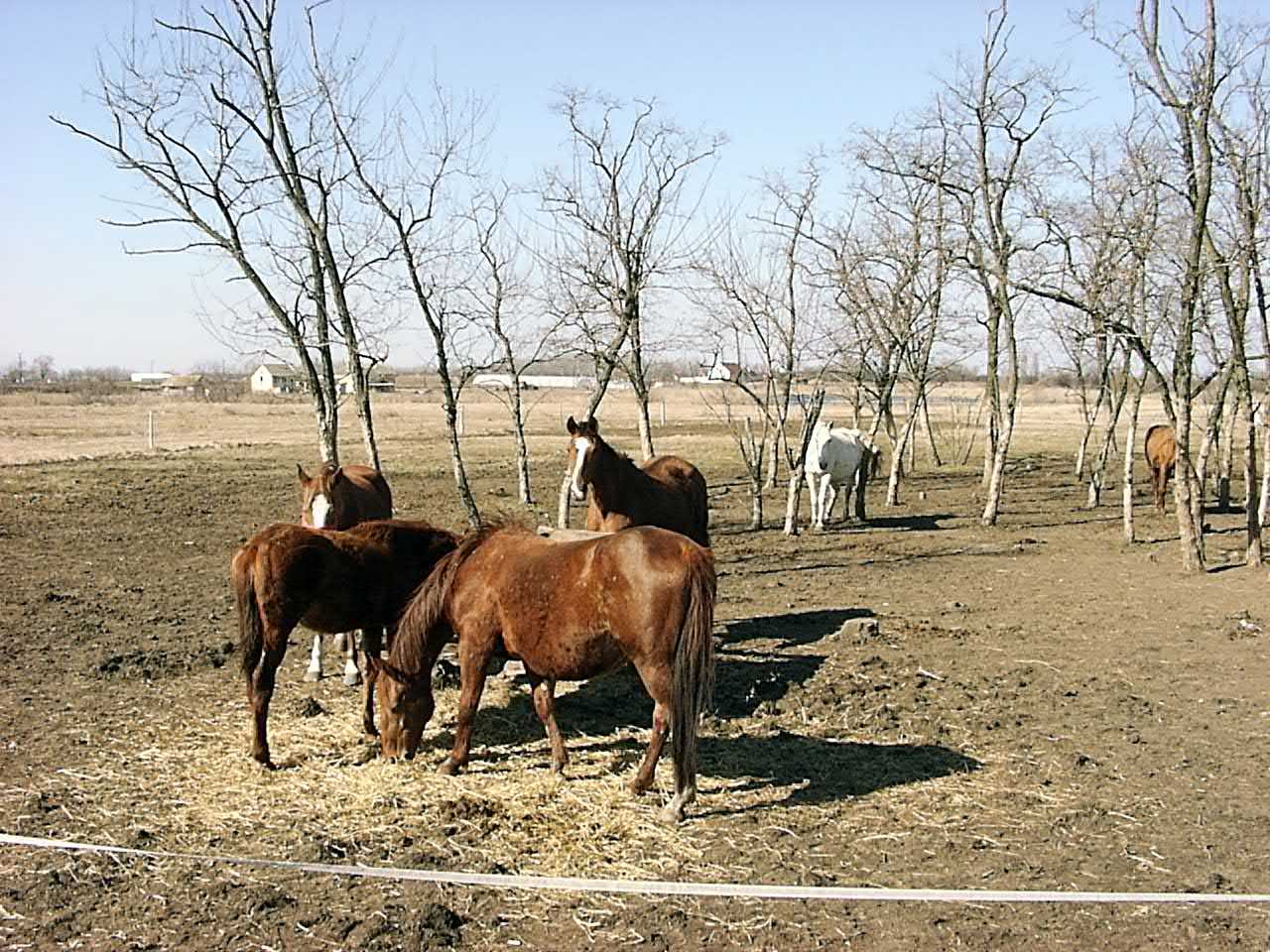The photograph captures a winter scene of a large, mostly barren farmland with sparse, short grass and mostly dirt. Central to the image is a group of four chestnut brown horses with white markings on their faces and brown manes, gathered around a pile of hay on the ground, with two of them actively eating. To the right of this group stands a white horse amidst a small thicket of bare, gnarled trees, facing the viewer. Further right, another brown horse, partially obscured, stands amongst more bare trees. A white horizontal strap, presumably a fence, runs across the lower frame, further indicating this is an enclosed area. The muddy ground consists of hardened clods of dirt with scattered hay. In the far distance, against a light blue sky with little to no clouds, there are several small white farmhouses and buildings. The few stumps in the area suggest recently cut-down trees. The entire scene is bathed in soft light, indicative of either late morning or afternoon.